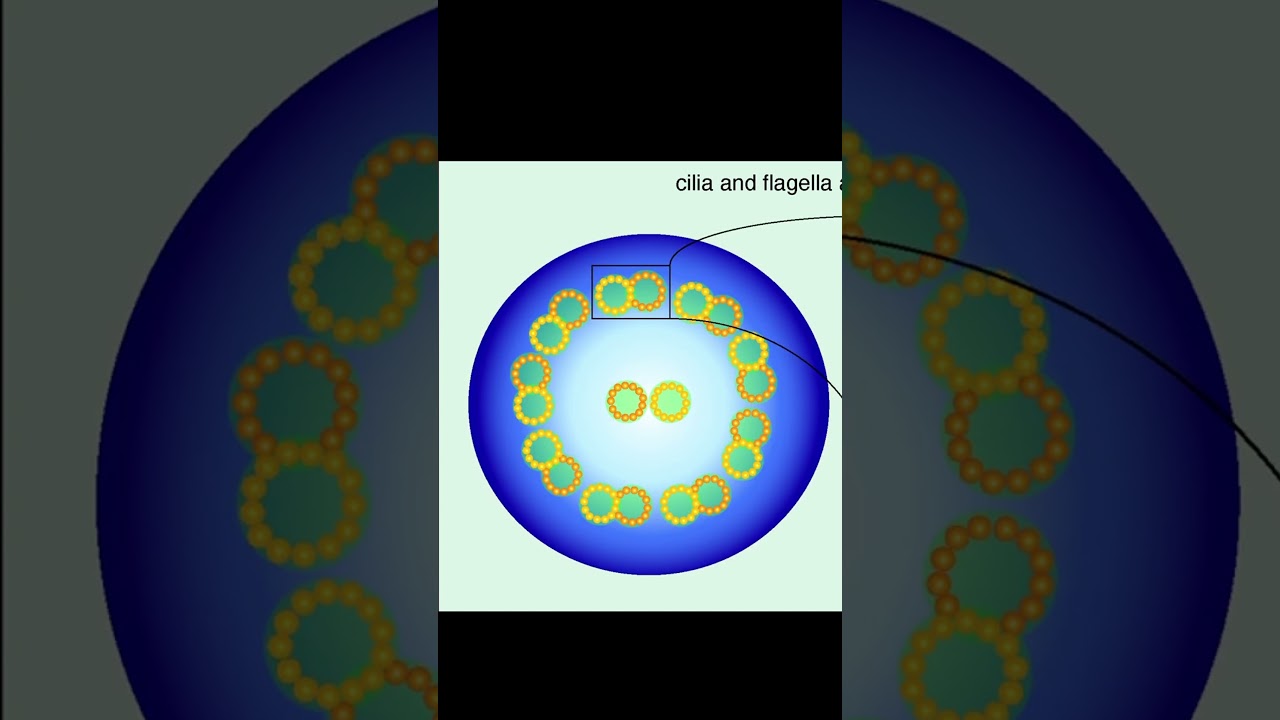The infographic presents a detailed and digitally rendered depiction of cilia and flagella. Central to the image is a small white box displaying a replicated view of a larger surrounding circle. This dominant circle, which has a dark blue gradient transitioning to a lighter hue in the center, contains numerous small gold, pearl-like rings that form a perimeter. Each of these rings encircles a green core, resembling tiny clustered pearls. Two of the gold rings within the larger circle touch, highlighted by a subtle green glow, while another pair of these rings sit separately in the center. The smaller, inset image also emphasizes this circular arrangement and is framed by a black border at the top and bottom, giving a defined contrast against its white background. Labeled "cilia and flagella," the inset box mirrors the larger circle but with finer detailing, including lines extending beyond, suggesting detailed connections. Despite the 3D intention of the graphic, it appears more like a gradient effect, adding depth, though not quite achieving a fully three-dimensional look.